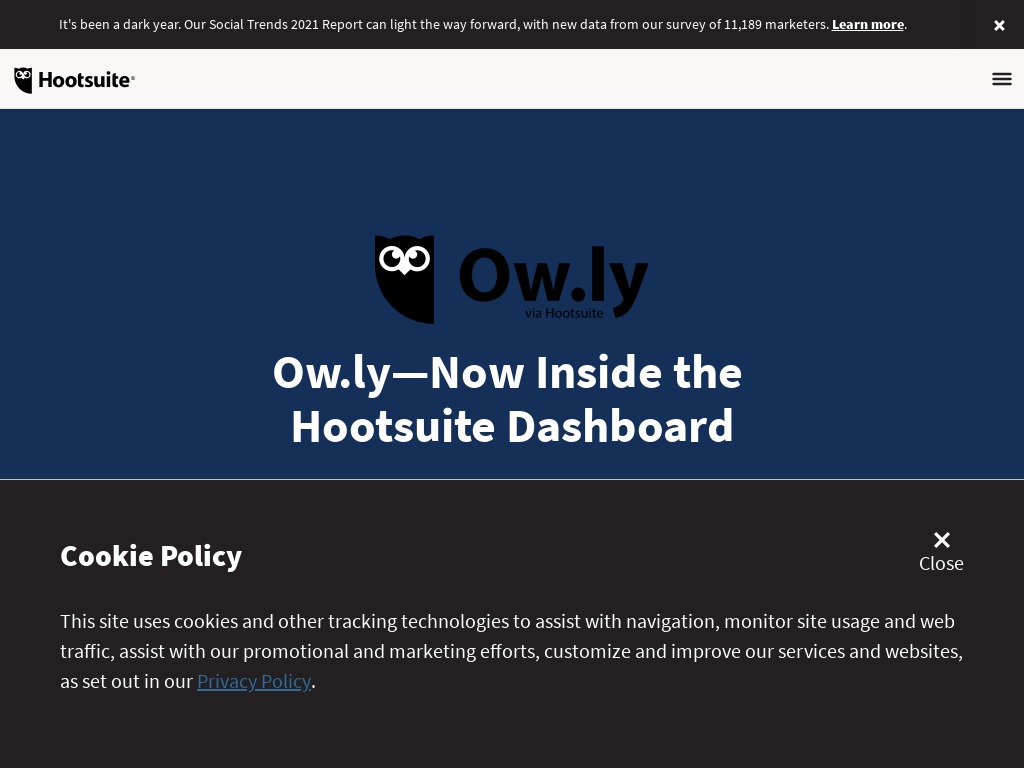Image caption: 
The image features a predominantly white background with a black box prominently displayed at the top. Inside the black box, bold white text reads, "It's been a dark year, our social trends 2021 report can light the way forward with new data from our survey of 11,189 marketeers." Below this message is a call-to-action link that says, "Learn more."

In the center of the image, the HootSuite logo is visible, consisting of the word "HootSuite" alongside a stylized owl within a semi-circle. Just beneath this, there is a navy blue box containing the word "Owly" and the same owl symbol. The text in the navy blue box reads: "Owly now inside the HootSuite dashboard."

At the bottom of the image, another black box contains white text detailing the site's cookie policy. The message indicates that the site uses cookies and other tracking technologies to assist with navigation, monitor site usage and web traffic, support promotional and marketing efforts, and customize and improve services and websites in accordance with their privacy policy. There is an 'X' in the top right corner of this black box, allowing users to close the message.